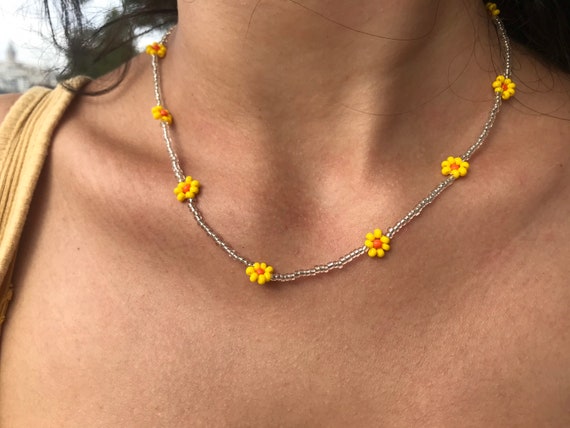The close-up image captures a woman's neck adorned with a delicate silver or clear-beaded necklace. This striking piece of jewelry features intricate yellow daisies with orange centers, spaced approximately every inch or two along the chain. There appear to be about eight visible daisies, suggesting a total of 10 to 12 flowers encircling her neck. The woman is dressed in a light yellow tank top, with a single strap visible over her dark brown or black hair, a few strands of which cascade down. Her skin is visible from the neck down to the top of her chest, with some veins subtly apparent. The background includes a slightly out-of-focus building, possibly a church or other large structure, along with a glimpse of the sky in the top left corner.